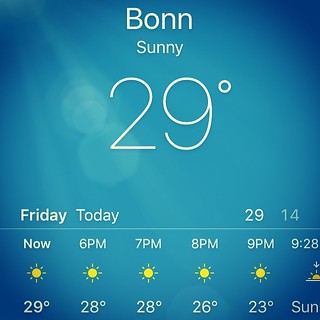A detailed, descriptive caption for the given image could be:

"In this vibrant weather app screenshot for the city of Bonn, the background features a gradient of blue hues transitioning from a darker blue in the corners to a brighter blue in the center, with artistic rays of light emanating from the upper left corner, creating a dynamic visual effect. At the top center of the screen, 'Bonn' is prominently displayed, followed by the word 'Sunny' beneath it. The current temperature dominates the display in large white font, reading '29°'. Below this, the app succinctly indicates today's date positioned to the left as 'Friday' and the temperature range '29° / 14°' to the right. A horizontal line divides the sections, leading to a timeline of weather forecasts: 'Now, Sunny, 29°', '6 PM, Sunny, 28°', '7 PM, Sunny, 28°', '8 PM, Sunny, 26°', '9 PM, Sunny, 23°'. Each time slot is marked with a yellow sun icon, signifying clear skies throughout the listed periods. Though partially cut off, the text '9:28' and 'Sundown/Sunset' can be discerned along the side of the screen. The overall color scheme of blue, white, and yellow creates a clean and visually appealing interface, emphasizing the clear, sunny weather in Bonn."